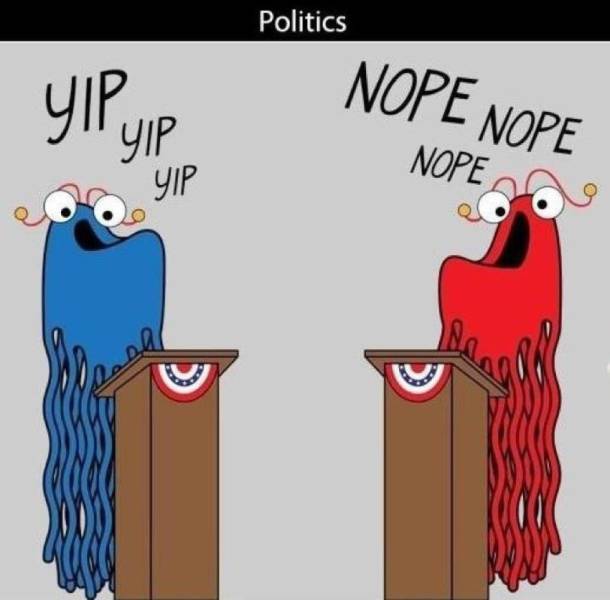The image is a cartoon meme satirizing politics. At the top, a black horizontal stripe bears the word "politics" in white lettering. Below, two blob-like monsters with tentacles for legs stand at podiums, facing each other. The creature on the left is blue and has large cartoonish white eyes, red antennas with yellow balls at the ends, and text above it saying "yip yip yip." The character on the right is red with similar features, but its text reads "nope nope nope." Both podiums are brown and adorned with a red, white, and blue semicircle flag on the front. The overall background is gray, emphasizing the contrast between the two opposing figures.